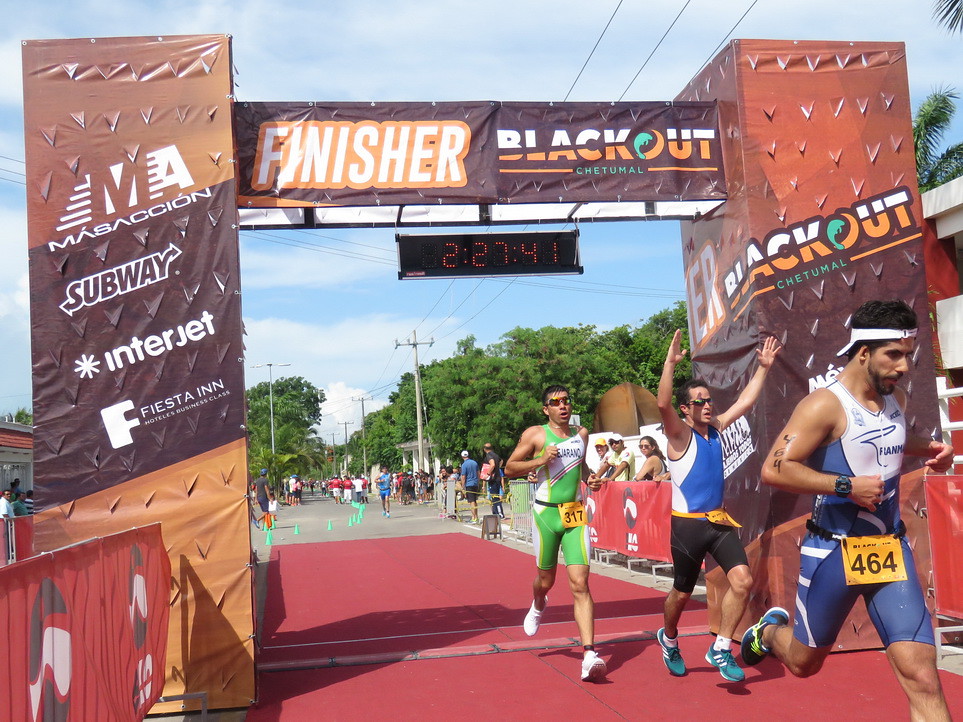This image depicts the vibrant and bustling finish line of a marathon, captured outdoors beneath a cloudy sky. Centered at the top of the image is an archway comprised of two square pillars supporting a banner that reads "Finisher Blackout Chetumal." A black clock with red lettering hangs from the middle of the archway, displaying a race time of 2 hours, 27 minutes, and 41 seconds. The archway and pillars exhibit a mosaic of colors, featuring shades of light and dark brown, white, and blue, and are adorned with sponsor logos, including Subway, Interjet, and Fiesta Inn.

In the foreground, three male runners clad in colorful running attire—green, white, black, blue, and red—are seen crossing a red carpet that covers the finish area. The athletes wear race bibs, with visible numbers 464 and 317. The runner on the right sports a backward visor, while the two behind him each wear sunglasses. Cones painted in light green line the path, enhancing the race's organized look.

Further back, more runners are approaching the finish line, alongside bystanders and volunteers who are lined up behind barricades. The backdrop features a mix of lush green trees and utility poles, contributing to the urban yet scenic atmosphere. The grey concrete street underfoot and the interplay of various colors create a dynamic and energized scene, emblematic of a well-organized marathon finish.